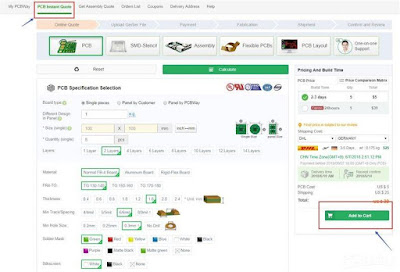The image is a detailed screenshot of an online PCB (Printed Circuit Board) order form from a website. At the top of the screenshot, you can see a navigation bar with several options, where the highlighted option is "PCB Instant Quote," indicated by an underline in orange, signifying it as the active page. Other visible navigation options include "Online Quote," "Upload Gerber File," "Coupons," and "Delivery Address," among others.

The main content of the form is prominently divided into two sections: the "PCB Specification Selection" on the left and the "Pricing and Build Time Summary" on the right. In the PCB Specification Selection section, the first row prompts the user for several essential details regarding their PCB order:

- **Board Type:** Options include "Single PCB," "Panel by Customer," and "Panel by PCBA Way."
- **Layers:** A drop-down menu offers choices such as "One Layer," "Two Layers," etc.
- **Quantity:** An input box where users can specify the number of boards needed.
- **Dimensions:** Separate input fields for entering the Width (in mm) and Length (in mm) of the PCB.
- **Board Shape:** Options include "Rectangular" and "Custom Shape."

Each category offers user-friendly interactive elements like drop-down menus and input boxes to facilitate the data entry process for the PCB specifications.